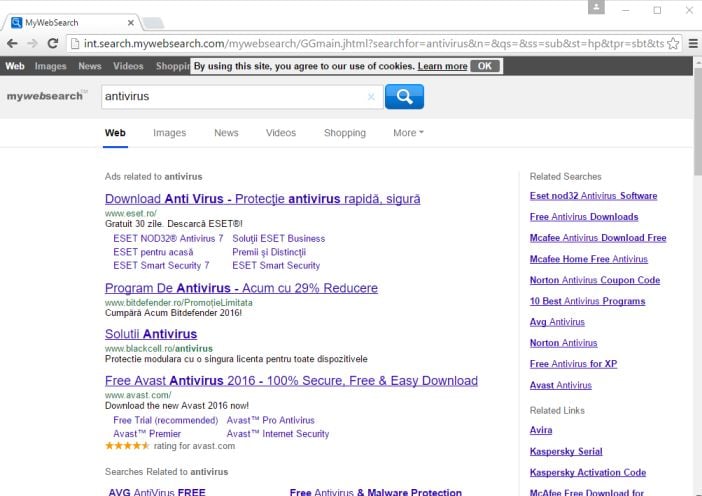This image depicts a "My Web Search" webpage with various search result categories, including Web, Images, News, Video, Shopping, and more, with the "Web" category highlighted in bold. Underneath the search bar, it appears that the word "antivirus" was entered into the search engine, returning a list of related search results.

The search results include:
1. **Download Antivirus - Protect Tile Antivirus Rapid**: A suggestion from Segura.
2. **Programa de Antivirus at a 29% Discount**: A result in Spanish from www.bitfinder.
3. **www.blackcell.ro/Antivirus**: Another option listed.
4. **Free Avast Antivirus 2016 - 100% Secure, Free, and Easy Download**: Promoted by Avast.com, emphasizing the availability of the new 2016 version.

Additionally, at the bottom of the search results, there are suggestions for related searches, including "AVG Antivirus Free" and "Free Antivirus and Malware Protection".

On the right-hand side of the webpage, there are approximately 15 related search items under "Related Searches", mentioning options like:
- **ESET NOD32 Antivirus**
- **Free Antivirus Downloads**
- **McAfee Antivirus Download Free**

Towards the bottom of the page under "Related Links", there are further suggestions for:
- **Avira**
- **Kaspersky Serial**
- **Kaspersky Activation Code**
- **McAfee Free Download**

These details provide a comprehensive overview of the antivirus-related content and suggestions offered by the "My Web Search" website.